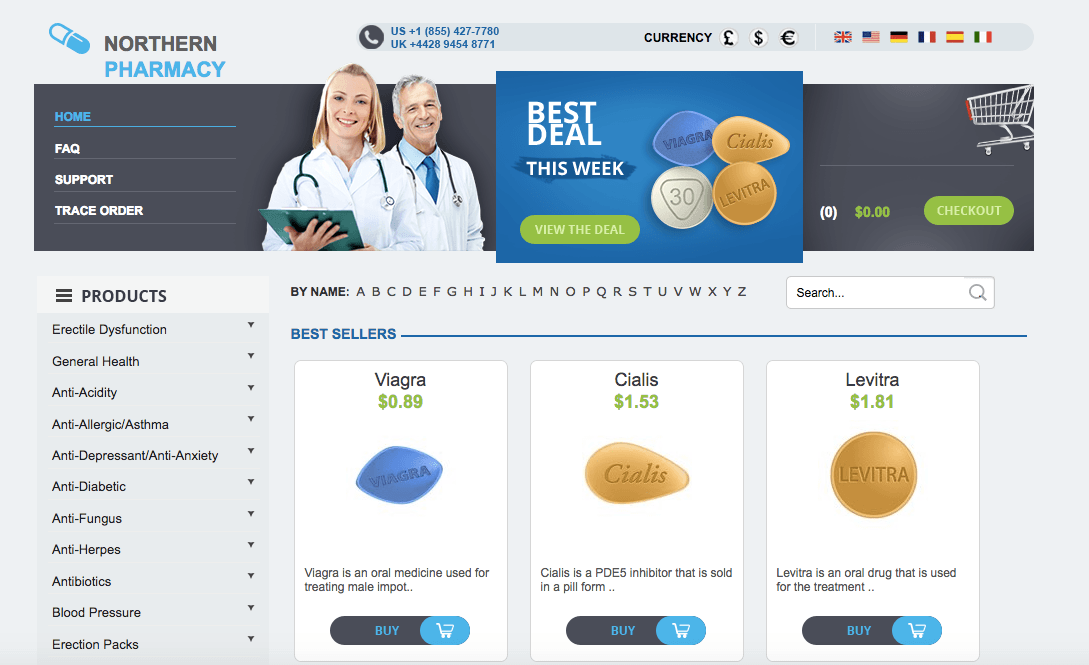The image features a banner with a black background running across the top. In the upper left corner, "Northern Pharmacy" is prominently displayed. Moving towards the right, there is a US phone number "1-855-427-7780" and directly below it, a UK phone number "+44 2894 548771." Further to the right, the word "Currency" is shown alongside symbols for the Pound, Dollar, and Euro. A series of flags, including British, American, and Italian, among others, are also present, though some are unspecified.

On the far left of the banner, a menu lists the following options in descending order: "Home" (highlighted in blue), "FAQ", "Support", and "Trace Order," all in white text. 

Adjacent to this menu, there are images of two doctors, one male and one female, both dressed in white coats.

In the center of the banner, a horizontally-oriented rectangle showcases a promotional feature titled "Best Deal This Week" with a call-to-action button labeled "View the Deals". Inside this rectangle, images of four types of pills are displayed: Cialis, Viagra, Levitra, and another unspecified pill.

To the right, there is an icon of a shopping cart with the text "Check Out" on a green button. The shopping cart shows "0 items" and "0 money."

Below the banner on the left side, a product menu lists various categories which have drop-down options: "Erectile Dysfunction," "General Health," "Anti-Acid," "Anti-Allergic," "Asthma," "Antidepressant," and "Anti-Anxiety."